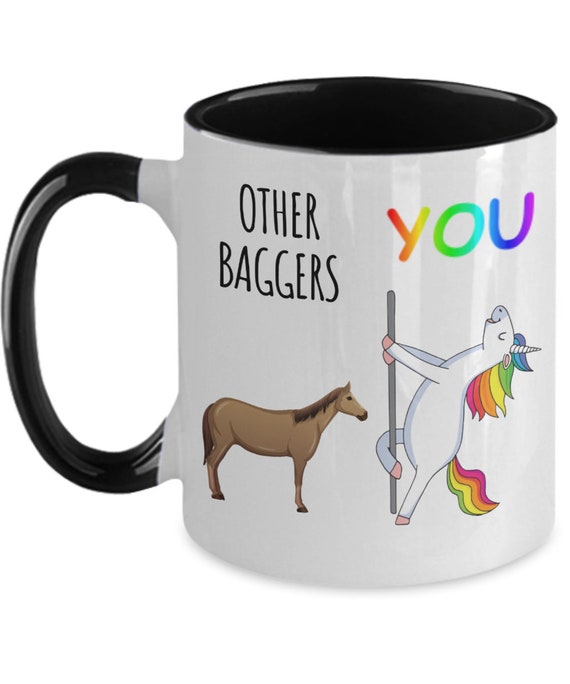The image showcases a white coffee mug adorned with a slender black handle and a black interior. Set against a white background, the mug features a whimsical design. On the right side, there's a brown, cartoonish horse with a brown mane and tail. Above this horse, in black letters, it says "Other Baggers." On the left side, dominating the scene, is a lively unicorn with a radiant rainbow mane and tail, sporting pink hooves and a joyfully expressive face. It clutches a pole in a pose reminiscent of a pole dancer. Above the unicorn, in vibrant rainbow-colored letters, it says "You." The overall contrast between the mundane brown horse and the colorful, exuberant unicorn adds humor and charm to the image.